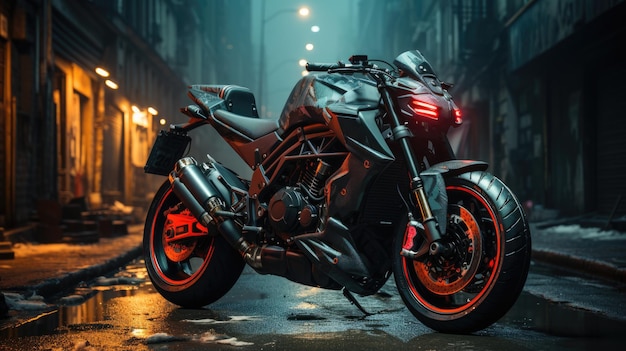This image features a CGI-generated red and black sports motorcycle prominently parked in the center of a wet, gray street, framed by buildings on both sides. The left-side building is adorned with small, warm yellow to orange lights that cast a soft glow onto the street below. At the back of the motorcycle, a series of at least five street lamps mounted on poles illuminate the scene, further contributing to the nighttime ambiance. The motorcycle itself has a striking design with red rims, a black seat, and four glowing red headlights, emphasizing its sporty aesthetic. The overall setting combines detailed urban elements with a focus on the central, vividly colored motorcycle.